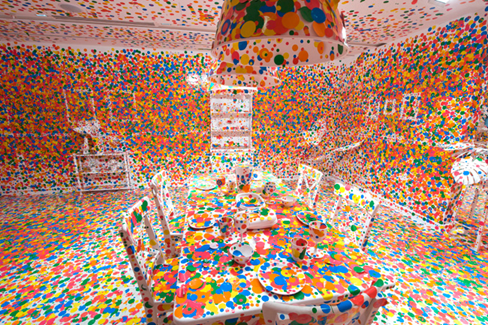The photograph captures a vibrant dining room engulfed in a kaleidoscope of colorful circles, creating a visually striking and festive atmosphere. Every surface in the room is meticulously adorned with dots in a spectrum of colors including blue, yellow, orange, red, green, and pink. These circles are omnipresent, covering the walls, ceiling, floor, and even the furniture with a certain thoroughness. The dining table at the center of the room, surrounded by four chairs, is also entirely covered in these multicolored dots, as are the plates, napkins, and other items on the table. The chandelier hanging from the ceiling is no exception, adorned both inside and out with circles. In the backdrop, despite the overwhelming dot pattern, one can discern shelves or doorways. The overall effect is reminiscent of a confetti explosion frozen in time, giving the room a lively party-like ambiance.